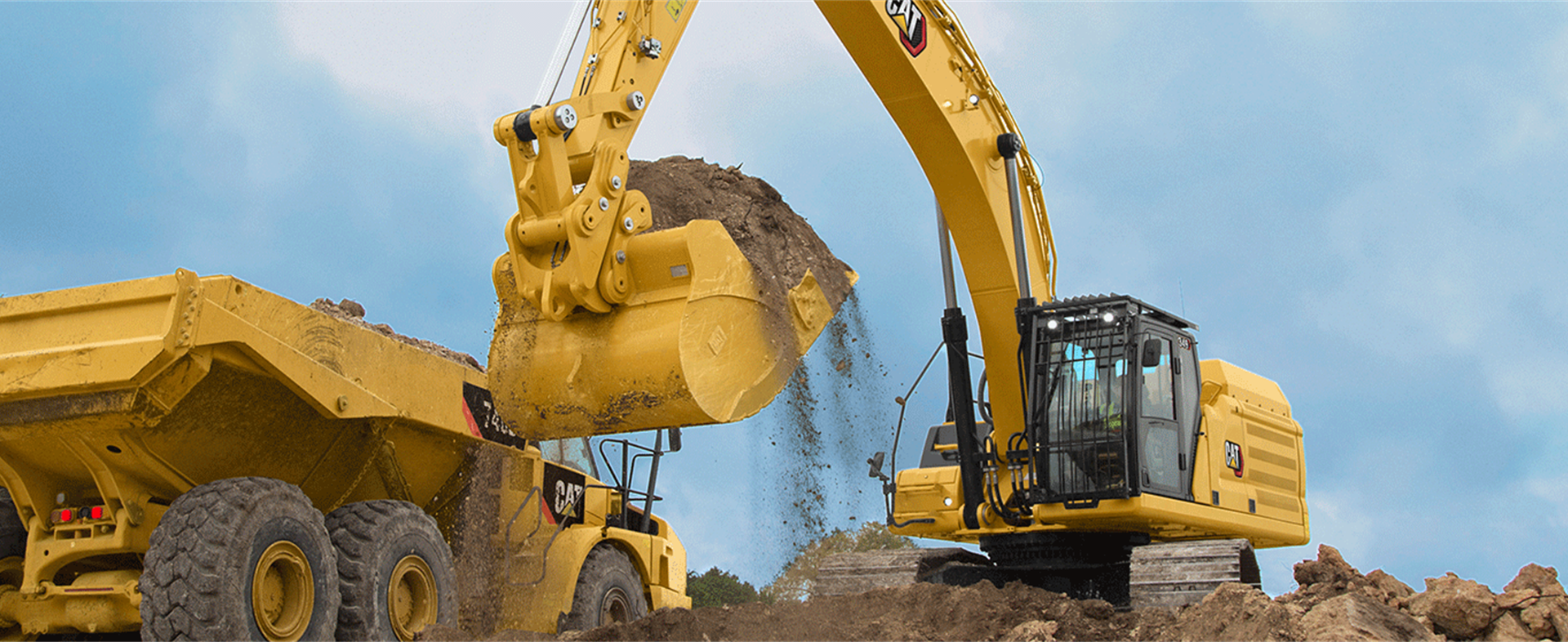The image depicts a bustling construction site under a bright blue sky. Dominating the scene is a large, yellow CAT backhoe, identified by its black CAT logo. This powerful machine, equipped with a long arm and a substantial shovel, is actively scooping up a massive load of dirt. The backhoe is in the process of depositing the dirt into the receptacle of a sizable yellow dump truck parked nearby. In the foreground, heaps of dirt and scattered boulders are visible, emphasizing the scale of the landscaping project likely aimed at leveling the land for a significant building endeavor. The photograph, captured in a horizontal, rectangular frame, encapsulates the industrious atmosphere of heavy machinery and determined construction efforts on a clear, blue-skied day.